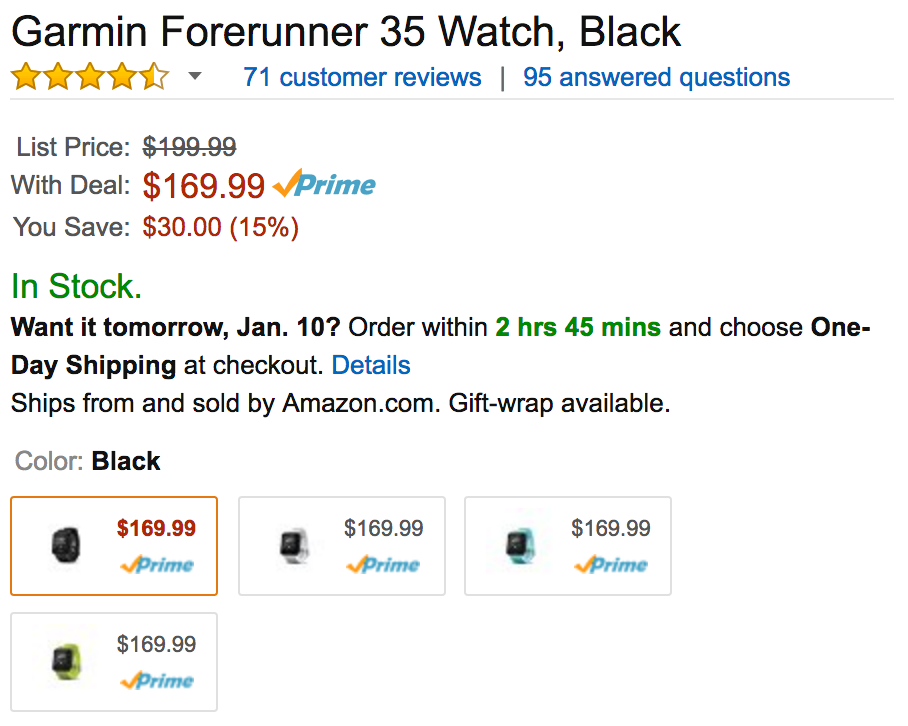Garmin 435 Watch in Black, Available on Amazon

Price: $199.00 
Price with Deal: $169.99 (Save $30, 15% off)

Prime Price: $169.99 

Availability: In stock 

Order by January 10th to receive the watch with 1-day shipping if you checkout within the next 2 hours and 45 minutes. 

Additional Details: 
- 71 customer reviews
- 95 answered questions
- Sold by: Amazon.com 
- Gift wrap available 

Don't miss out on this Prime deal for the Garmin 435 watch in black, offering essential features at a discounted price. Get it now for $169.99 and enjoy swift delivery with Amazon Prime.